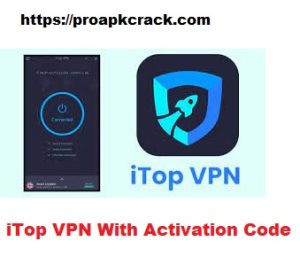Screenshot of a web page with a white background. At the top, the URL "https://proapkcrack.com" is displayed in black text. Below the URL, there is a centrally positioned turquoise box containing two images. The image on the left depicts a mobile phone screenshot with a prominent blue "on" button in the center. The image on the right shows an icon representing a VPN service; it features a black background with a blue shield icon containing a rocket in the middle. Beneath this icon, the text "iTopVPN" is written in blue. Outside the turquoise box, the phrase "iTopVPN with activation code" is displayed in red. The rest of the screenshot features a white background with substantial spacing between the URL at the top and the turquoise box in the center.